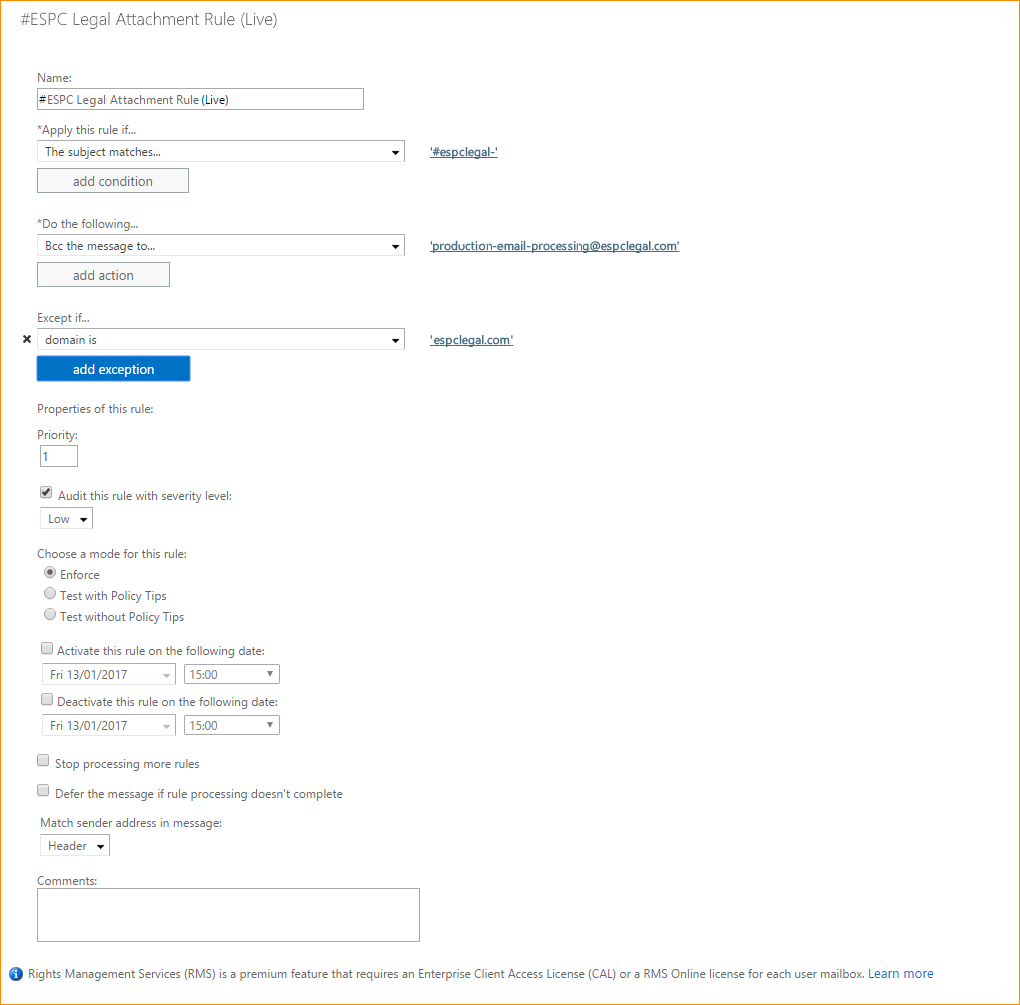**Detailed Caption:**

This square-format, color image illustrates the user interface of a dry and purely functional computer-generated form, specifically designed for setting rules in an application.

At the top left of the form, the label reads "#ESPC Legal Attachment Rule," indicating the purpose and context of the settings. Below this, the user is presented with fields to fill in, beginning with the "Name" field, which has already been populated with the same label, "#ESPC Legal Attachment Rule."

The form is structured to follow a conditional logic layout, resembling a flow chart. The first actionable option is "Apply this rule if," followed by a dropdown to select conditions like "the subject matches," allowing the user to specify criteria for applying the rule. Users can add multiple conditions as needed.

Next, the form states, "Do the following," with the initial action set to "BCC the message to...," accompanied by an input field where the user has specified a recipient. This action details the automatic blind copying of messages under the rule's conditions.

Further customization includes an "Except if" clause, which allows the user to define exceptions for when the rule should not be applied, adding another layer of specificity.

Additional fields include "Properties of this rule," which lists attributes such as priority and an auditing requirement marked with a severity level of "Low." It also presents a "Mode" dropdown with options like "Enforce," "Test with policy tips," and "Test without policy tips," among which "Enforce" is selected to implement the rule actively.

The overall design, while not visually appealing, emphasizes functionality and clarity for users setting conditional rules within the application.